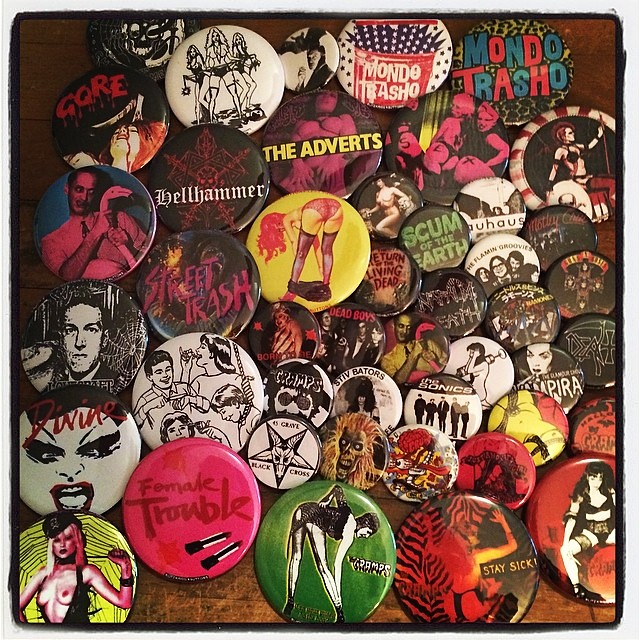The image depicts a diverse collection of punk rock pins scattered across a wooden table against a whitish background. Each pin features unique and vibrant designs associated with the punk and rock scenes, boasting a range of colors including white, black, brown, blue, yellow, pink, purple, and various shades of gray. Notable pins within the collection include ones for the bands Bauhaus and the Ramones, both positioned on the right side of the table, as well as multiple pins for the Kramps, one for Guns N' Roses featuring artwork from "Appetite for Destruction," and another for Motley Crue. Additional pins carry names and graphics like "Street Trash," "The Adverts," "Mondo Trasho," "Stay Sick," "Scum of the Earth," and one with the band members of the Sonics. A distinctive pin featuring a topless woman is found in the left corner. The display appears to be a snapshot of a personal collection, reflecting a strong rock and punk aesthetic.